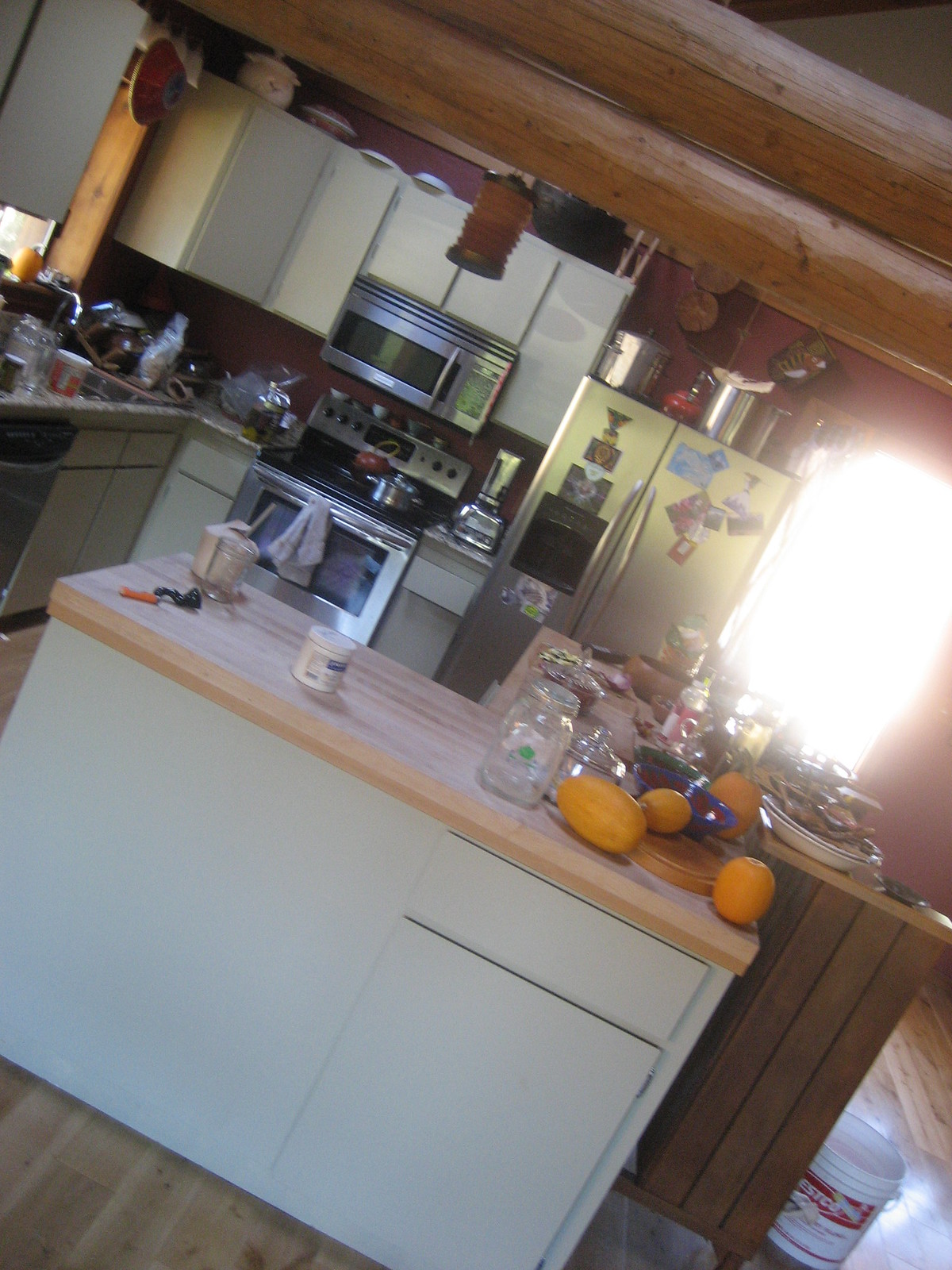The photograph captures a bright and spacious kitchen bathed in daylight. At the center of the room stands a white kitchen island with a wooden butcher block countertop, adorned with a couple of oranges, a mason jar, and a glass dish. A stainless steel refrigerator, decorated with magnets and family photos, occupies one side of the kitchen, with pots and pans stored on top. Nearby, an oven and stove are visible, a silver pot resting on a burner and a dish towel draped over the oven handle. A blender is positioned beside the stove. 

White cabinets line the walls, providing a clean and classic look, while the wooden floor adds warmth to the space. A white plastic bucket with a red label sits on the floor. The sink area shows some dishes stacked on the counter, and a jar of pickles is placed beside the oven. Wooden beams on the ceiling add a rustic touch to the room. The presence of sunlight streaming in through unseen windows enhances the inviting atmosphere of this well-used and loved kitchen.